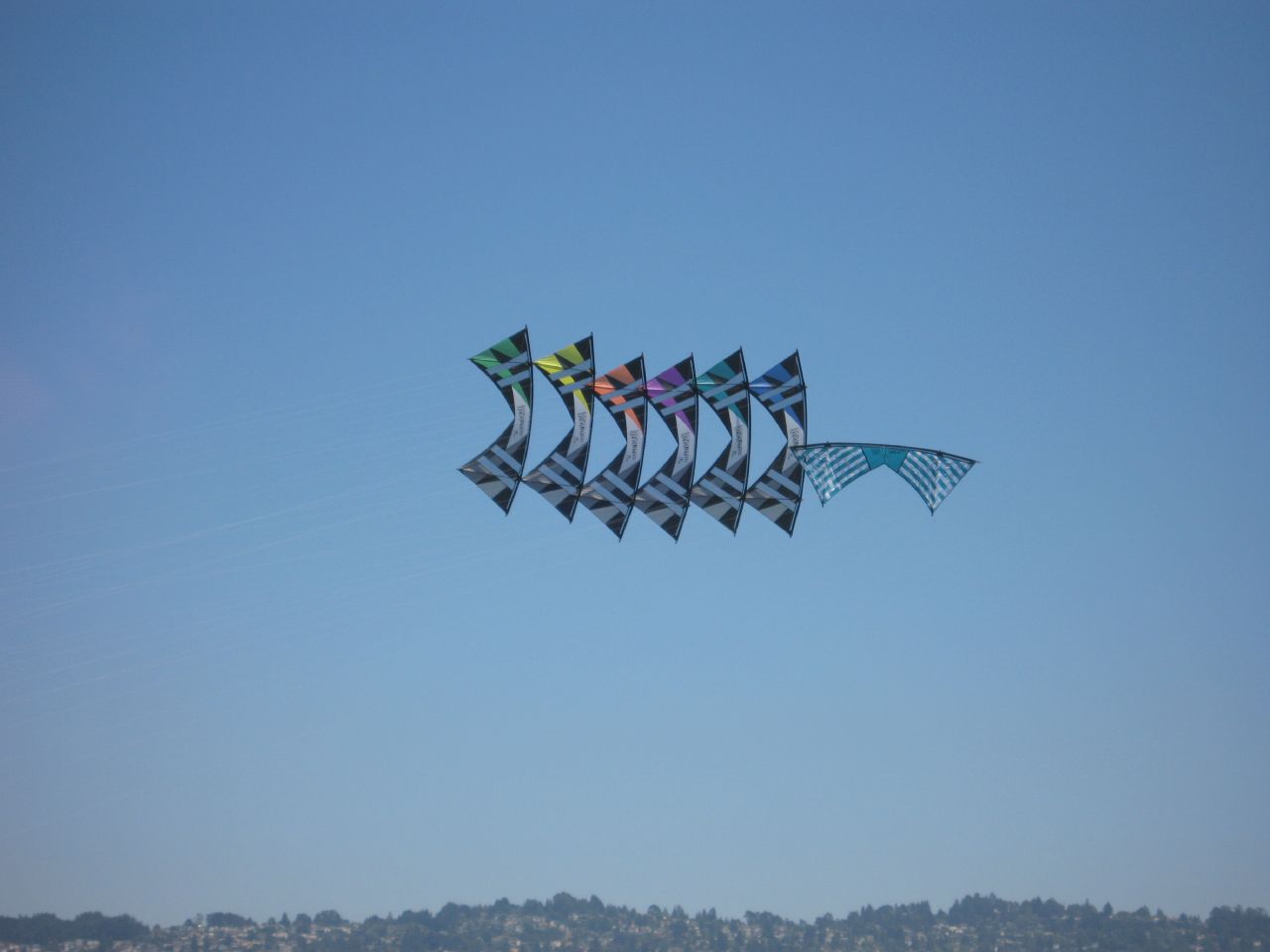In this photo, captured from the ground with the camera angled upwards, a bright, light blue sky without any clouds forms the backdrop. At the bottom of the picture, far off in the distance, there's a tree line featuring various types of vegetation, but the details are indistinguishable. Dominating the middle of the image, soaring in the sky, is a colorful series of kites strung together in a vertical arrangement, resembling bow ties connected at their ends. Each section of the kite has its own distinct color schemes: starting from the right, there is an all-blue kite, followed by a blue and black one, another blue and black, then a purple and black, an orange and black, a yellow and black, and finally on the far left, a green and black kite. The kite sections are designed with vertical and horizontal lines, adding to the vibrant display against the mostly clear sky. Despite the slightly fuzzy quality of the photograph, the intricate patterns and colors of the kites create a striking visual centerpiece.